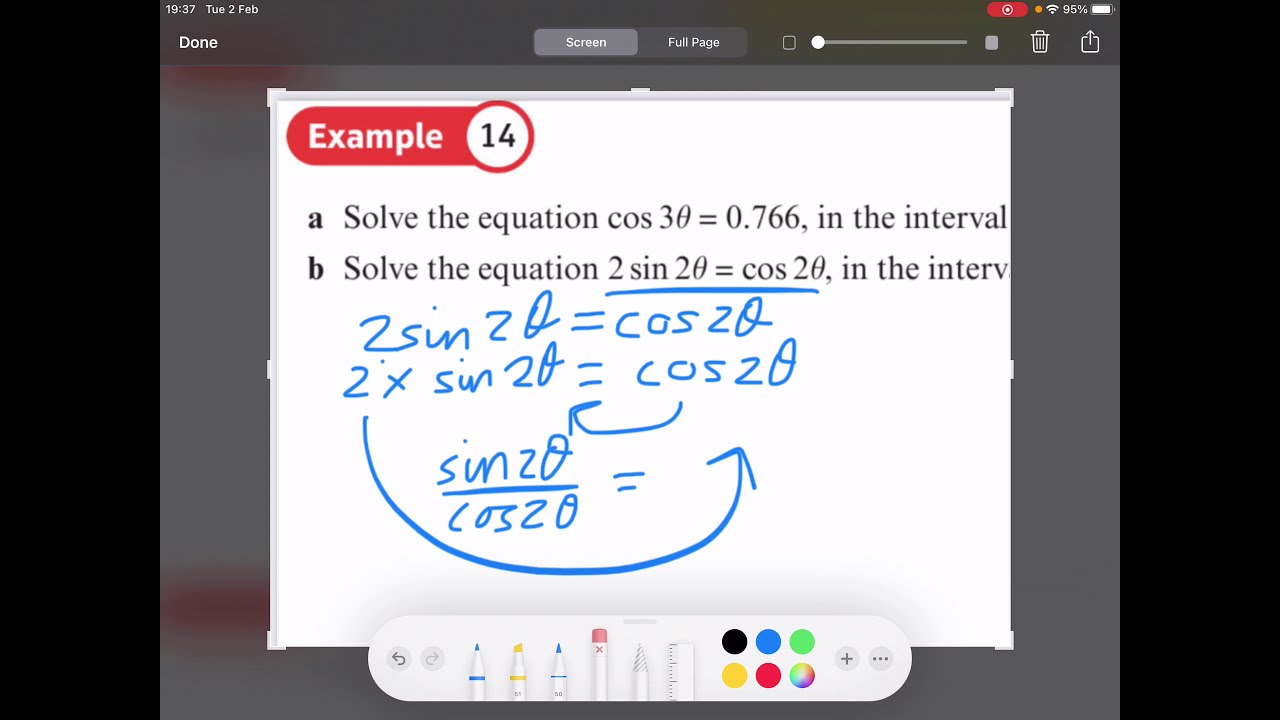This image is a horizontally aligned rectangular screenshot of an online exam page displayed on a computer or tablet screen, bordered by thick edges on either side. The screen's background is gray, featuring toolbar icons at the top, such as a play button, a trash can, and a share button, along with options labeled "screen" and "full page". The top-left corner indicates the date and time as Tuesday, February 2nd, 19:37, alongside Wi-Fi and battery status icons. Central to the gray background is a square white page with "example 14" written in red at the top. Below this heading, two math problems are listed, labeled A and B. Problem A instructs to solve the equation "cosine 3θ = 0.766 within a specified interval," while Problem B presents the equation "2 sine 2θ = cosine 2θ within a specified interval." Handwritten solutions in blue are displayed beneath each problem, demonstrating the work. Additionally, there are editing tools below the problems, indicating options for different types of pens, colors, and sizes, suggesting the use of a photo editor.